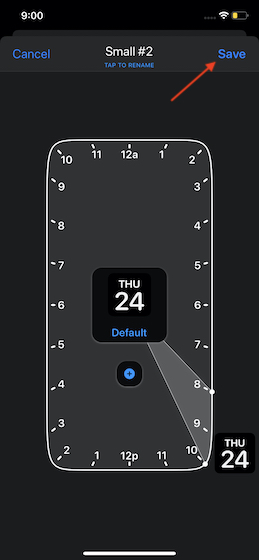This is a detailed screenshot of a digital clock display, captured from a mobile application with a minimalist design. The status bar at the top left shows the current time as 9 o'clock, while the top right features icons indicating Wi-Fi strength and battery life, with the battery indicator nearing the low-power red zone but still orange.

At the very top of the screen, there are navigation and action buttons: "Cancel" on the left and "Save" on the right, both highlighted in blue. Positioned centrally is a header that reads "small world number 2," and beneath this is a blue text prompt: "tap to rename."

The main clock interface, which utilizes a 24-hour format, is dominated by a black circular face displaying the current day, date, and a default label. The specifics are: Tuesday, 24th, which appears in white text in the upper arc of the circle. The "default" label at the bottom of the circle stands out in blue. Just below this circle is a blue plus button, likely intended for adding new entries or settings.

Encircling the clock interface is an external black bubble overlaying the phone or watch face, reiterating "Thursday, 24th" in white text. The overall background color of the application is black, enhancing the contrast and readability of the digital elements.